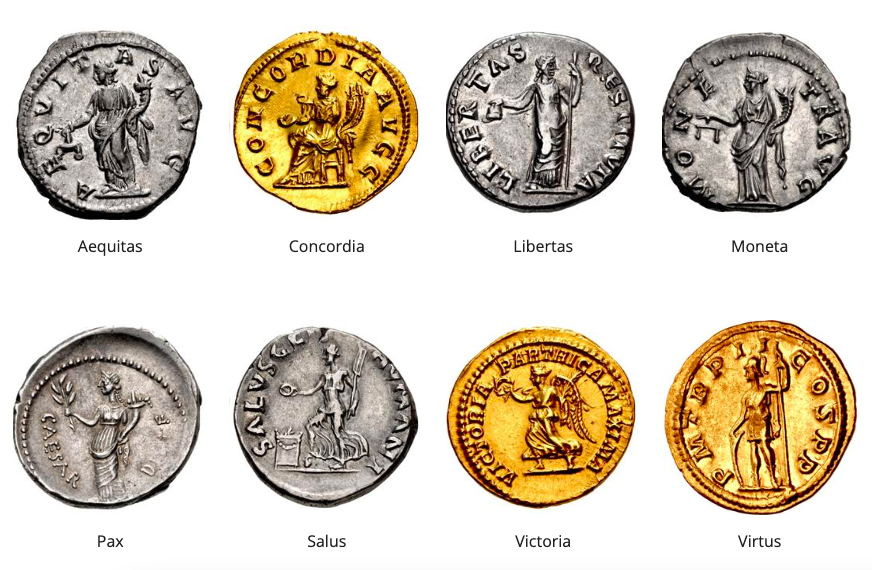The image showcases a detailed arrangement of eight distinct coins against a white background, organized into two horizontal rows of four coins each. These coins, with an ancient, Greek-inspired design, display noticeable imperfections in their roundness, suggesting they were likely stamped by hand rather than modern machinery. Each coin features the image of an individual engaged in various activities, contributing to their uniqueness. The coins vary in color, with a mix of silver and gold hues. Underneath each coin, the inscriptions read Equitas, Concordia, Libertas, Moneta on the top row, and Pax, Salus, Victoria, Virtus on the bottom row. The text appears in clear, although slightly blurred letters for some names, positioned beneath their respective coins. The overall style and presentation of the image evoke a historical or archaeological vibe, reminiscent of an old coin collection.